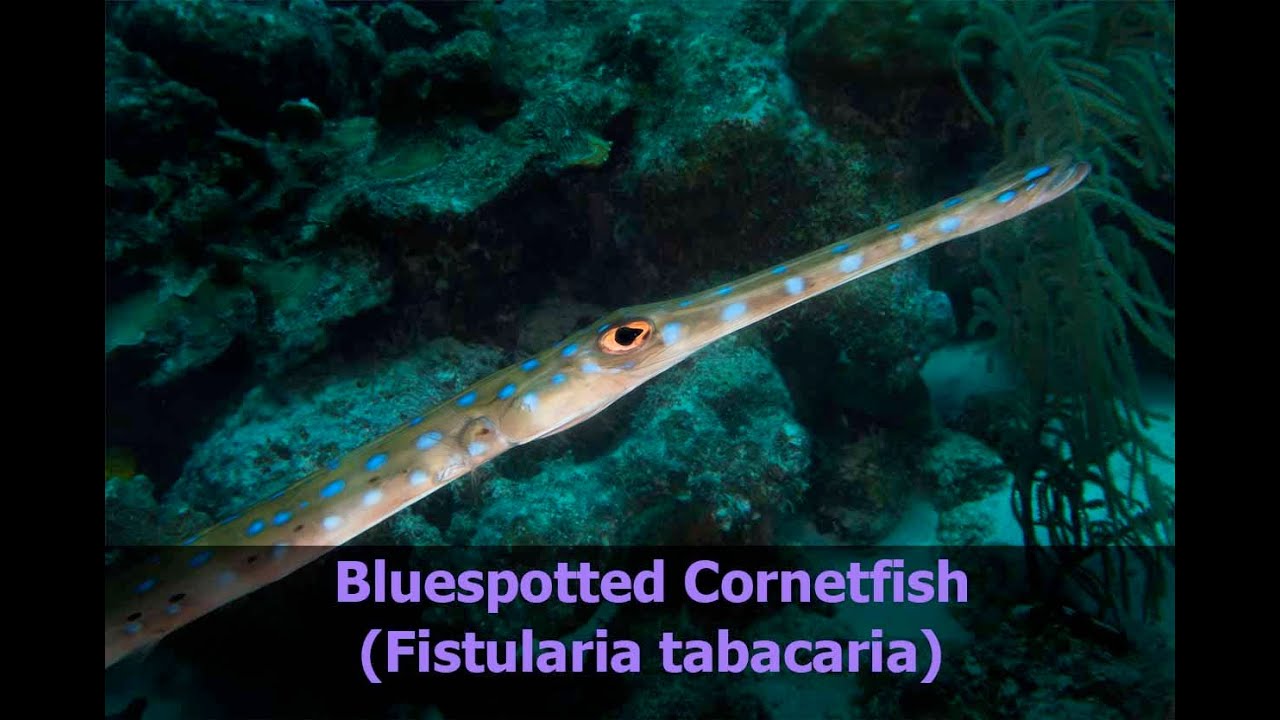This underwater photo features a striking blue-spotted cornet fish (Fistularia tabacaria), distinguished by its elongated, snake-like body and long, crocodile-like snout. Its coloration is unique: the top half of its body is green, transitioning to a beige underside, and it is adorned with blue polka dots running along its length. The fish has distinctive yellow-orange eyes with black pupils. It is swimming in a vibrant undersea environment, where the left side of the image is dominated by sharp, green coral formations, while the right side includes clusters of green plants. The sand at the bottom of the photo appears white but is tinted green due to the underwater light. A transparent text bar with purple lettering identifies the fish and its scientific name.